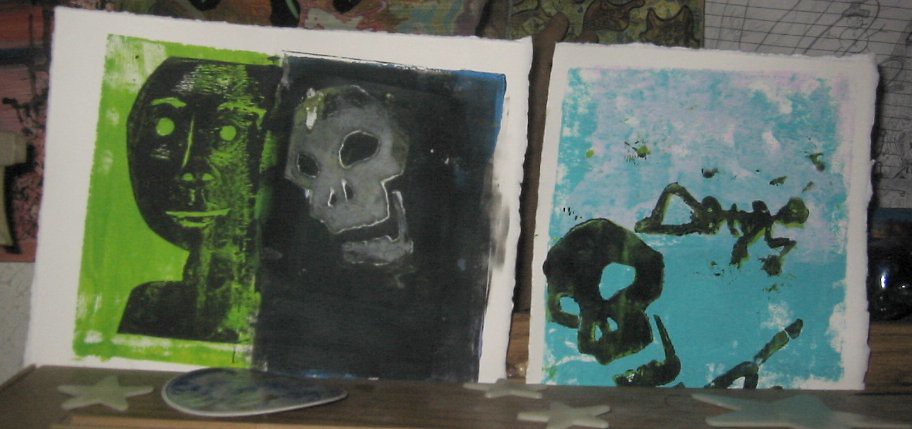The image depicts an exhibit showcasing a table with diverse geometric objects and paintings. Prominently displayed on the table are several three-dimensional stars, varying in size and shades of gray, scattered across its brown surface with one notably larger star on the right. On the left side of the table lies a disc or rounded object, face-up. Behind these objects are two vertically positioned paintings, each bordered in white. 

The painting on the left, rectangular in shape, features two distinct sections: the upper half displays a green background with a cut-out silhouette of a bald human figure, the features (eyes, nostrils, lips, and eyebrows) cut out to reveal the green background beneath. The lower section presents a black background with a gray skull. The second painting, square and positioned to the right, showcases a blue background, prominently displaying a black skull in the bottom left corner and some black graffiti-like lines extending from the bottom right. There is also text in the middle of this painting which appears to read "Dave" or "Doyle."